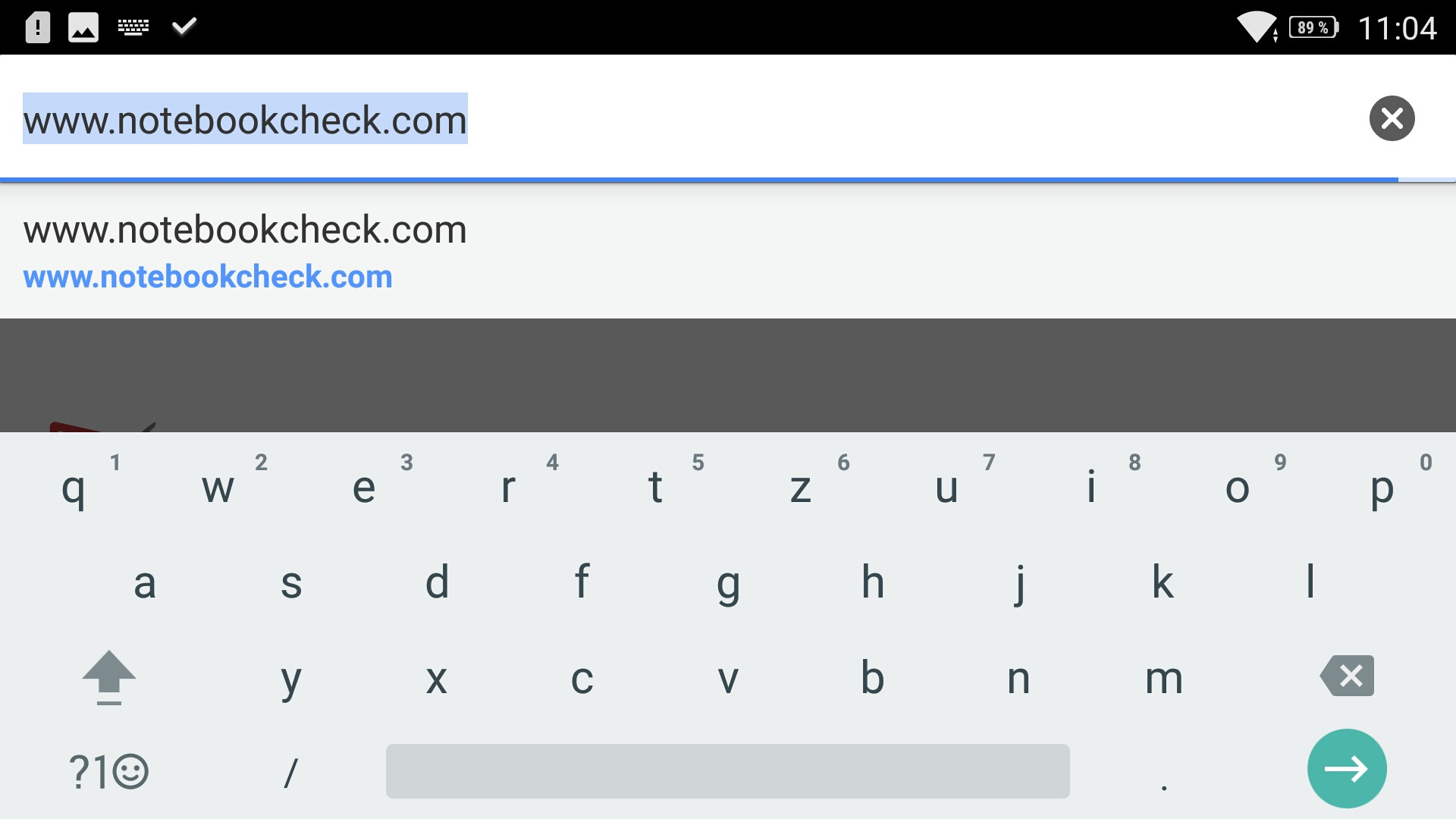The image captures a screenshot from a cell phone browser displaying the website www.notebookcheck.com. The top of the screen features a light blue rectangular border on the left-hand side, enclosing black-font text. On the same horizontal line, towards the far right, there is a grey circle containing a white 'X'. Directly below this, a thin blue line spans the width of the screen. Below the blue line, a darker off-white box extends from left to right, again showing the URL www.notebookcheck.com. Underneath, the URL appears once more in blue text: notebookcheck.com. Further down, a darker grey bar extends across the screen from left to right. At the bottom, the virtual keyboard is visible, with black keys displaying numbers and letters spanning the full width of the screen.